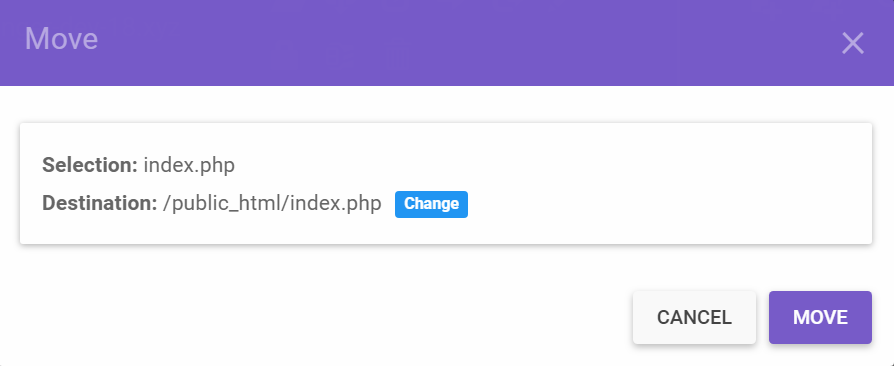In this image, we see a long, rectangular, purple box extending horizontally across the top of what appears to be a screenshot. Inside this box, the word "Move" is displayed in light lavender text. At the far right end of the purple box, there is a small "X". Below this is a lightly gray rectangular box containing black text. Within this gray box, the text "selection: index.php" is bolded. Directly beneath this, the bold phrase "destination: /public_html/index.php" is visible. Adjacent to this phrase, there is a blue box with white text that offers the option to "Change". At the very bottom right corner of the image, there are two more boxes: a white box with the word "Cancel" and a purple box with the word "Move".